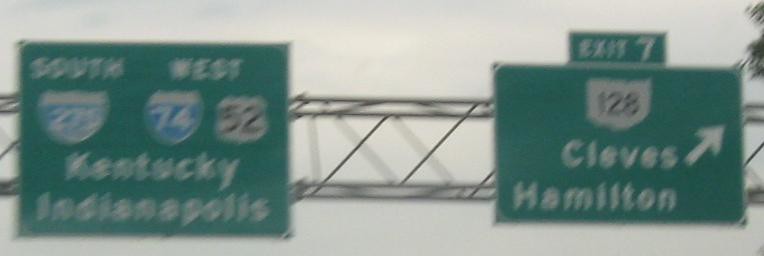In this detailed highway sign image, we observe two significant signs directing drivers. The larger sign on the left is green and square-shaped and is designed to guide travelers moving south and west. At the top of this sign, in white lettering, "South" is displayed on the left and "West" is on the right. Directly beneath these directional indicators, the numbers "275," "74," and "52" are prominently shown, representing major highways. Further down, the sign contains the names "Kentucky" and "Indianapolis" in clear white text.

To the right of this main sign, there's a smaller, rectangular green sign. At its very top, "Exit 7" is written in white text, indicating an upcoming exit. Below this, the sign features the number "128" in black text on a white background. Further down, the name "Cleves" is displayed, with an arrow pointing to the right to guide drivers. Just beneath "Cleves," the name "Hamilton" is listed.

The signs are mounted on a black overhang structure, providing a sturdy base for their display. The sky in the background is a light gray, contributing to the overall visibility and clarity of the signs for drivers.